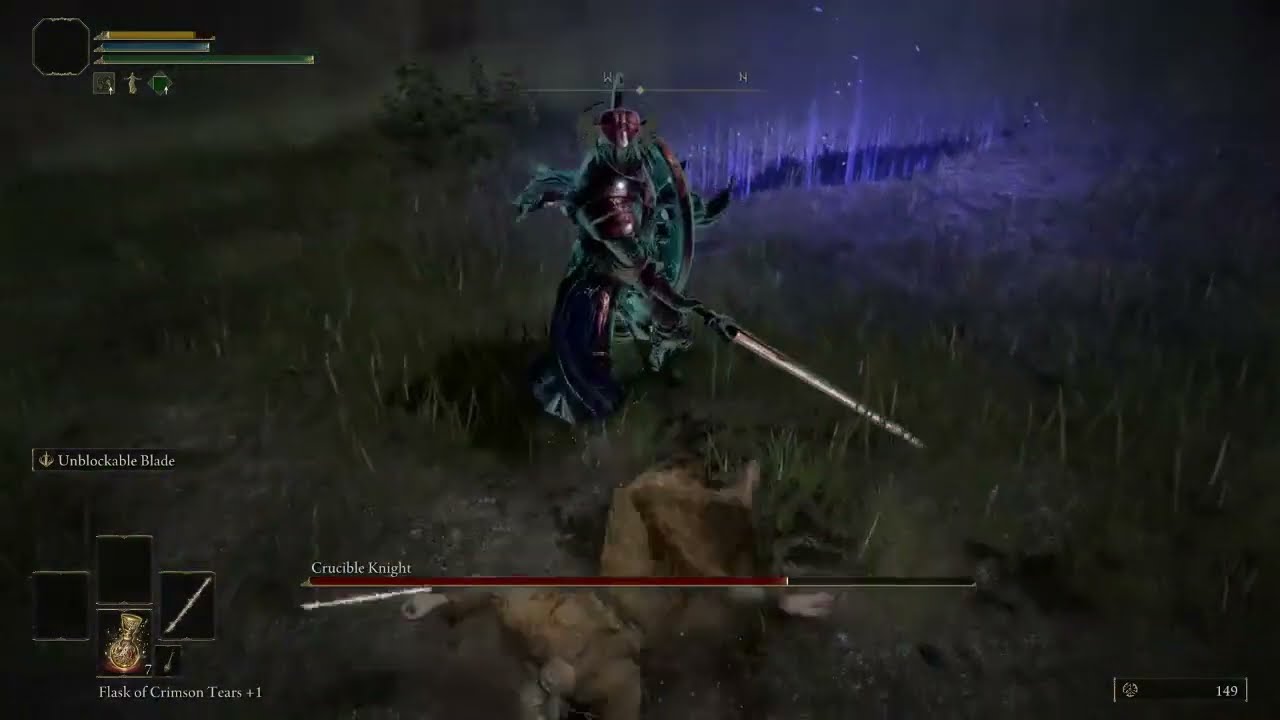This full-color digital image, horizontally rectangular and relatively dark in tone, captures a dramatic scene from a computer game. The setting appears to be an outdoor field, possibly during rain, marked by the dim hues of browns, greens, and subtle touches of blue and red. At the center of the image, a warrior known as the Crucible Knight lies fallen on the grassy ground, clad in brown robes. Standing over him is another knight, garbed in samurai-like armor, poised mid-swing with a long sword highlighted in white. This victorious knight faces the viewer, his sword creating an action streak towards the right side of the image. Notably, the ground to the knight's right is cracked, from which bright, blue rays and embers emanate, adding to the mystical atmosphere. The lower left corner of the image displays in-game awards such as a "flask of crimson tears +1" and an "unblockable blade" option. The upper left corner is filled with gauges indicating power and strength levels, contributing to the game's interface elements.